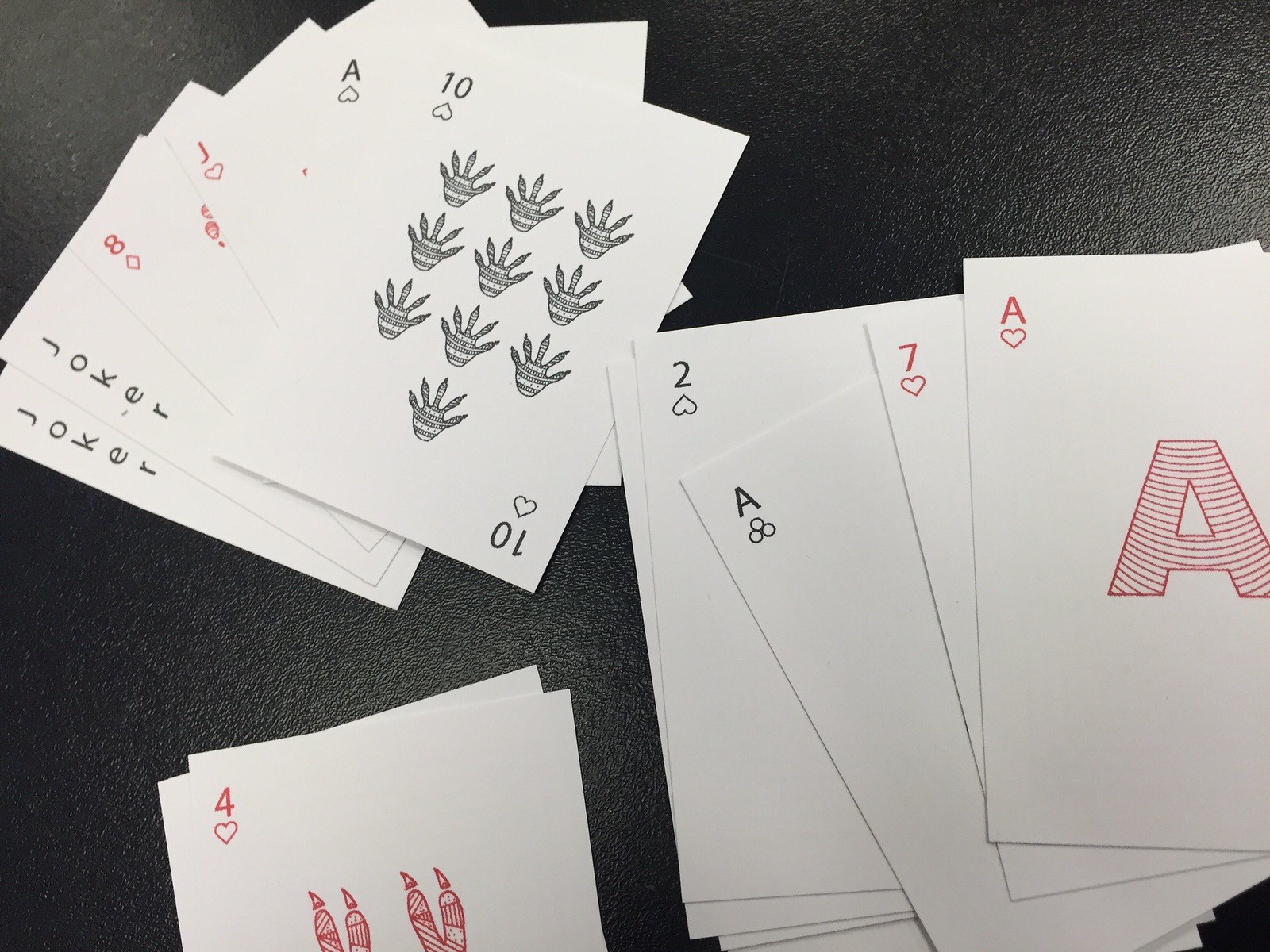The image features a collection of playing cards organized into distinct piles, each showcasing unique and unusual illustrations. 

In the upper left corner of the image, one pile of cards is slightly fanned out, revealing the faces of several cards. The visible cards in this pile are two Jokers, the Eight of Diamonds, the Jack of Hearts, the Ace of Hearts, and the Ten of Hearts. The Ten of Hearts is particularly notable for its distinctive illustration: a black and white sketch depicting a bird's foot with five toes, adorned with horizontal stripes.

Beneath this pile, another pair of cards is partially visible. The top card is the Four of Hearts, featuring a small sketch of pointy toes with sharp fingernails. The card beneath it remains obscured and indistinguishable.

To the right, there is another pile containing the Eight of Hearts, Seven of Hearts, Ace of Clubs, and Two of Hearts. Among these, the Ace of Hearts displays an illustration of a simple letter "A" embellished with swooshy lines drawn in red ink.

All of these playing cards are laid out on a sleek, black plastic table, adding a modern contrast to the traditional playing card designs with their whimsical and unconventional artwork.